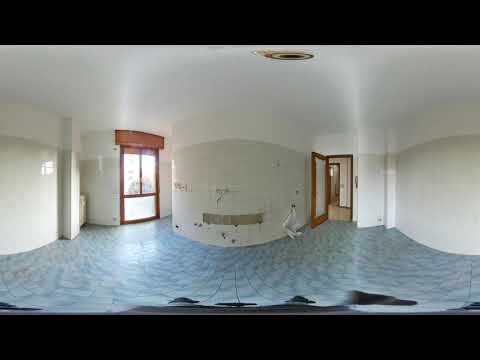This photo captures an empty, slightly disorienting room, likely due to the fisheye lens used, which gives the image a curved, broad view. The room, rectangular and vertical in orientation, features white walls and a white ceiling. The floor is tiled with a blue material, possibly resembling a tarp or wavy ocean-like blue tiles. There's a long, floor-to-ceiling window on the left, framed with dark brown wood, and an open wooden doorway on the right. Some details are fuzzy due to the image's quality, but a significant section of the wall appears damaged, with wiring exposed, possibly from something having been previously mounted there. At the top center of the ceiling is a circular object with concentric designs in black, white, and wood colors. Horizontal black bars appear across the top and bottom of the image.